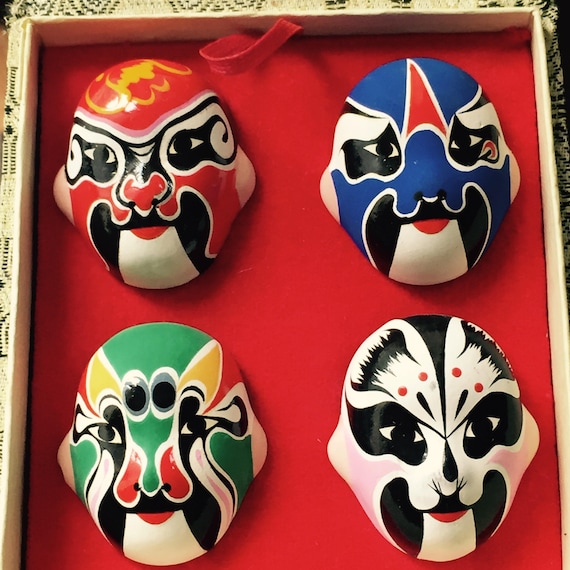The image showcases four ceramic or plaster masks, each painted in a unique palette but sharing a similar design. Arranged in a small, shallow box lined with bright red fabric, the masks are adorned with fluid, wavy patterns. The top left mask combines red, gold, black, and white, while the top right features red, blue, black, and white hues. The bottom left mask is the most colorful with green, yellow, red, black, pink, and white, and the bottom right mask is predominantly white with black, red, and pink accents. Each mask's eyes are painted black, with intricate designs surrounding them, adding depth and character. These vibrant masks are perfectly framed against the red background, further highlighted by a delicate doily placed behind them, making them a striking display of creativity and artistry.